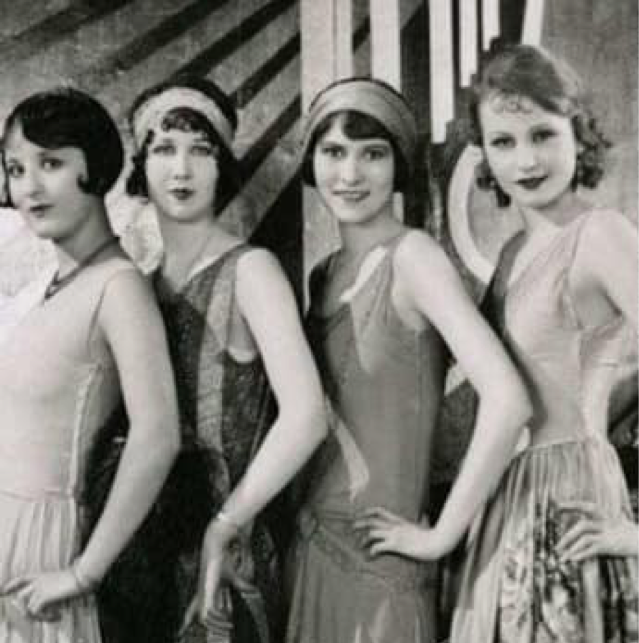In this black and white photograph from the 1920s, four young flapper women are captured standing in front of what appears to be a mural or poster featuring shadowed stripes. Dressed in long, form-fitting, flowy, sleeveless dresses with lower bust lines, they exude the iconic flapper style. Each of the women has short hair – three with varying styles of black hair, and one with light brown or blonde hair. The middle two women sport large headbands. All four have thick lipstick, and their hairstyles and attire reflect the fashion of the era. They stand in a confident, unified pose, each with their left hand resting on their left hip, and all except one, who showcases her teeth, smiling with their lips. Their slight tilt towards the viewer, combined with the intricate backdrop, captures the essence of the 1920s flapper look.